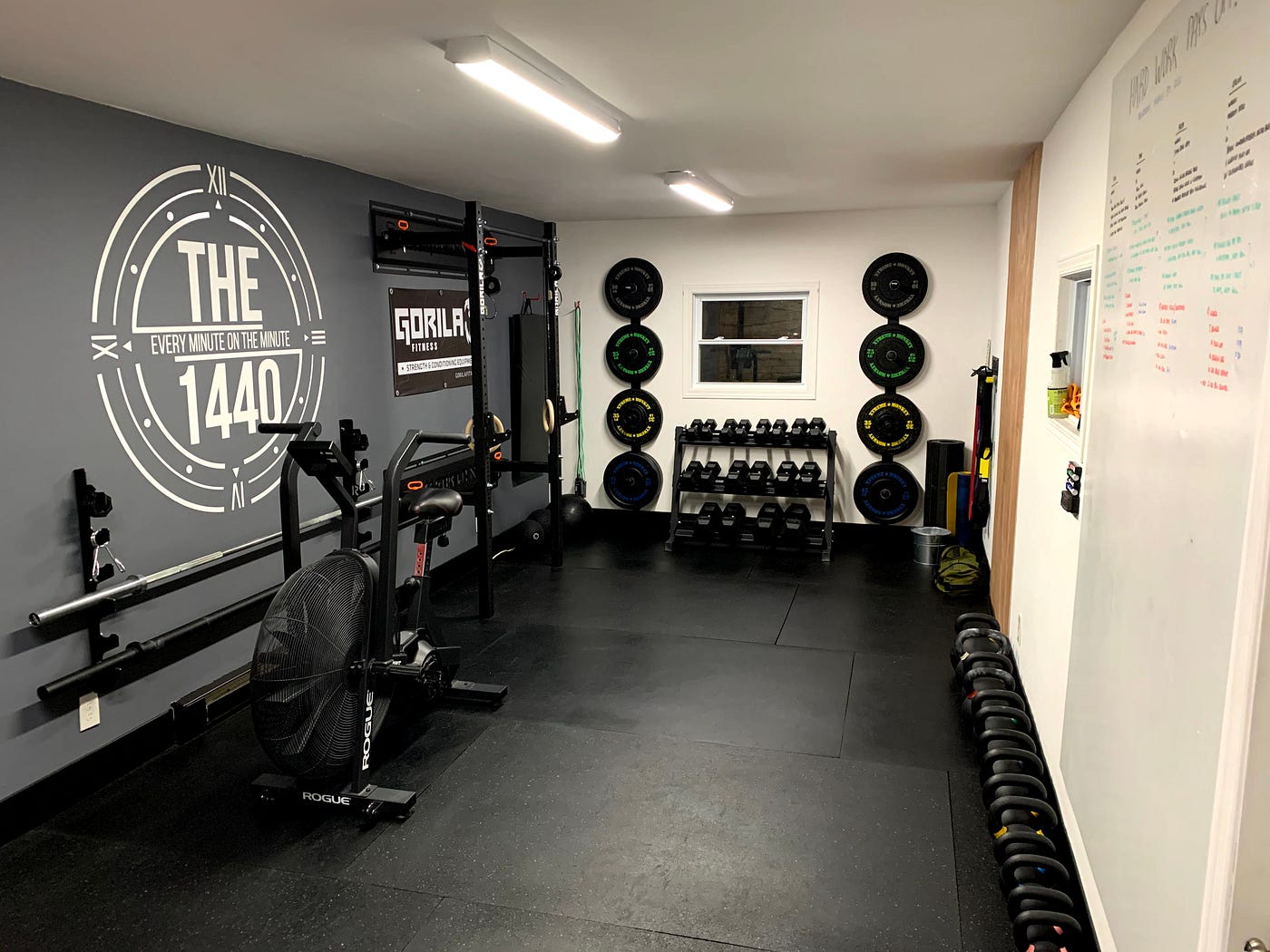This image depicts a weight room with a detailed and well-organized setup. The room features a black floor and is surrounded by walls of varying colors. On the left wall, which is gray, there is a prominent white circle containing the text "THE, every minute on the minute, 1440" as well as another sign that reads "Gorilla Fitness." Directly in front of this wall, near the back of the room, there is a squat rack and a cycling machine.

The back wall of the gym is white and features two vertical columns of weights, each comprising four rows. There is also a weight rack against this wall, with various dumbbells neatly organized beneath a small window. Additional weights, including kettlebells, are positioned on the floor.

On the right wall of the gym, there is a large whiteboard that extends from the ceiling to the floor, covered in notes and drawings in black, green, and red sharpie. Below the whiteboard, there are kettlebells and a small window housing some cleaning solutions. This side of the room also contains various exercise equipment such as bands, and a trash can situated nearby.

Overall, the weight room is compact but efficiently arranged, with clear areas for different types of workout activities and ample equipment for users.